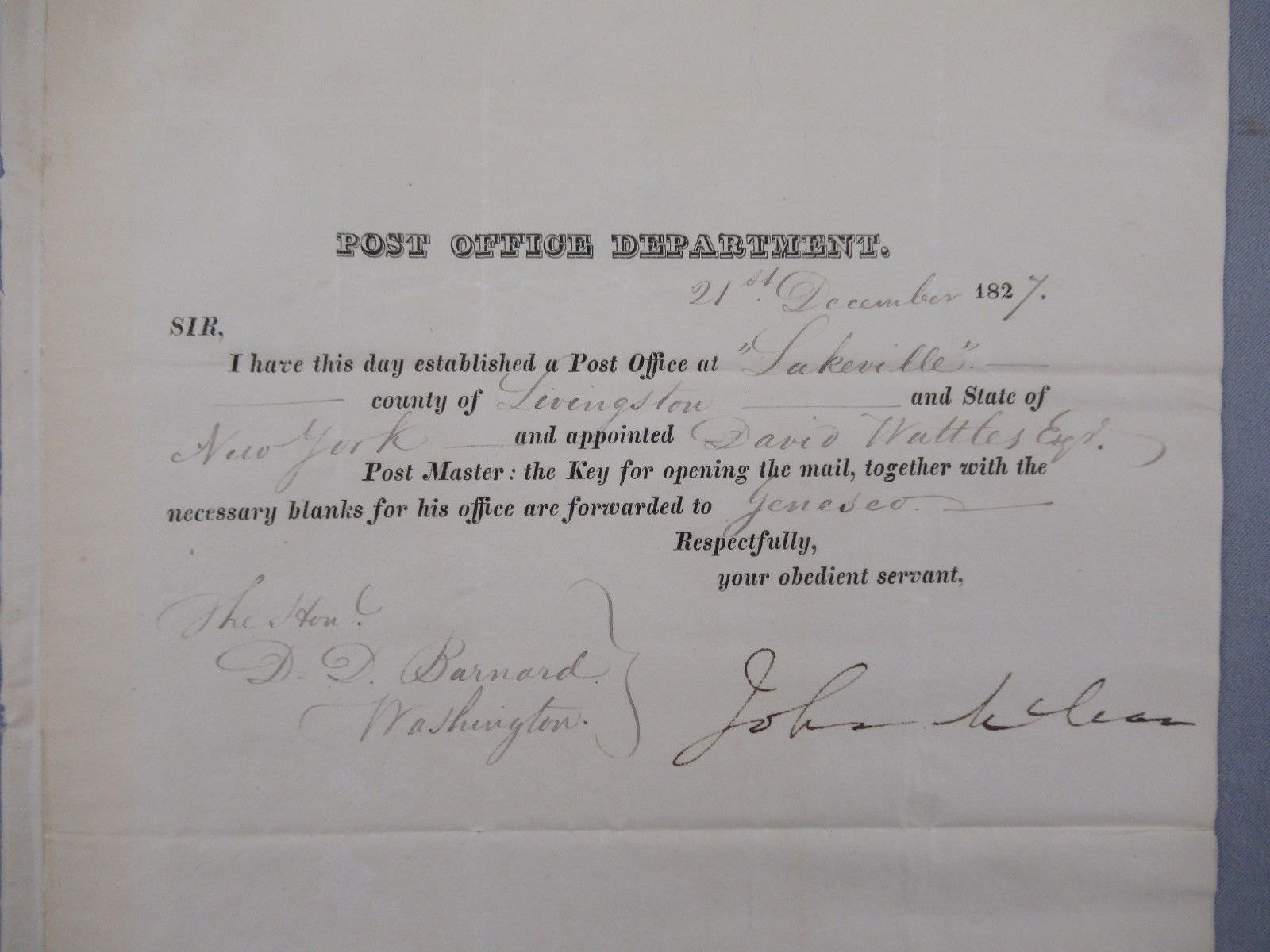This photograph captures a historic document from the Post Office Department, dated December 21, 1827. The piece of paper, marked with stamps indicating its age, announces the establishment of a post office in Lakeville, County of Livingston, State of New York. It states that David Wattsfield has been appointed as Postmaster. The note includes a combination of typed and handwritten text, with the latter being in cursive and somewhat difficult to read. At the bottom, there are multiple signatures written in cursive, appearing on the left and right corners. The document details that the key for opening the mail, along with the necessary blanks for the office, have been forwarded to Geneseo. The white background of the image contrasts with the aged appearance of the paper.